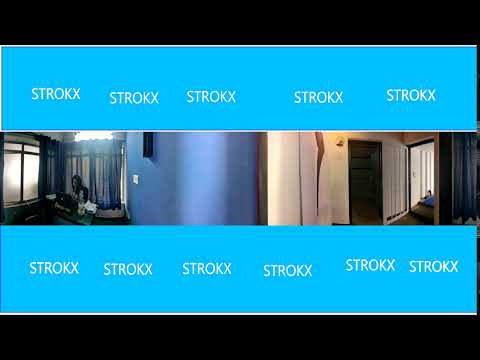The image in question is a 360-degree panoramic interior shot of a room or apartment. The image is bordered by a bright blue frame with white text that reads "STROKX," repeated five times at the top and six times at the bottom. Additional black rectangular frames form a letterbox effect at the top and bottom of the image.

In the scene itself, a woman is sitting at a desk on the left side, intently working on a computer. Behind her, a window with a blue curtain is visible, along with a large blue wall adjacent to her. To the right of her, the interior leads into a hallway with white walls. The hallway, which features a black doorway and wooden floors, extends into another, unseen room. On the right-hand side of the image, there are shadows and the presence of a mirrored door, adding to the detailed spatial context of the room.